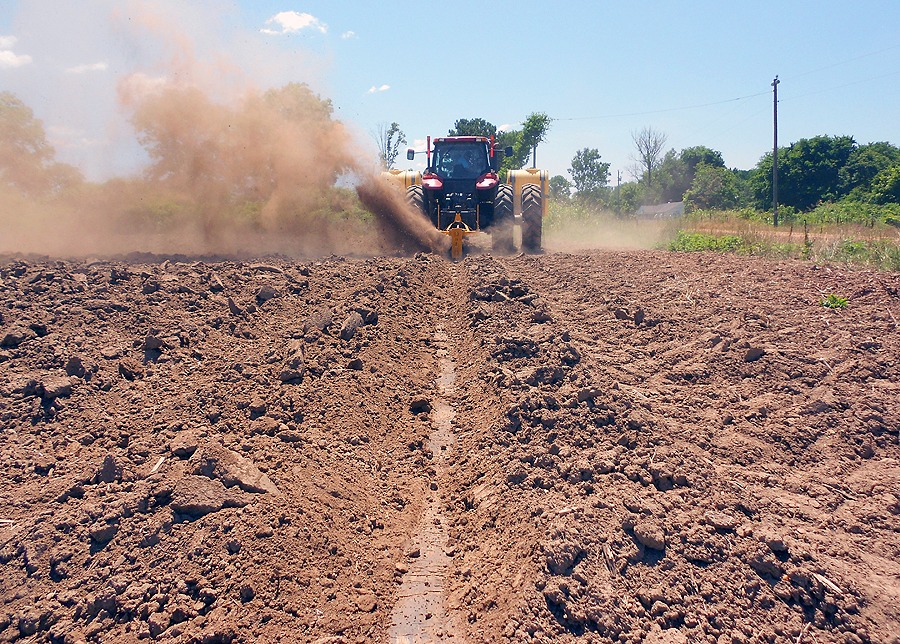The image captures a dynamic scene of a large, reddish-colored tractor with four prominent wheels as it advances towards the viewer, methodically tilling the soil. In the foreground, freshly plowed rows of soil extend towards the tractor, creating a visible path of overturned earth from the bottom of the photo. This action generates a substantial dust cloud that lingers in the air, emphasizing the machine's powerful movement. The tractor, accompanied by two yellowish tanks with grayish-black accents attached to its sides, is the central focus amidst an expansive dirt field or farmland. Above, the bright blue sky and a backdrop of trees and grass frame the scene, indicating it is a clear, sunny day. The photograph exudes a sense of agricultural labor and the vigorous activity of soil preparation.